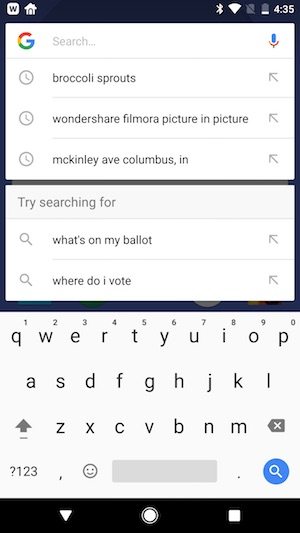This is a detailed screenshot from a smartphone. In the upper left corner, there is a black banner featuring a white square with a black "W" inside. Adjacent to it is a white house icon. On the right side of the banner, various status icons are visible: a Bluetooth symbol, a network signal indicator, a battery icon, and the number "435."

Below this banner, the background is entirely white. Prominently displayed is a multicolored "G" symbol representing Google. Beside it, in pale gray letters, the word "search" is visible, accompanied by a blue and orange microphone icon.

Underneath, the section labeled "suggested searches" lists the following queries: "broccoli sprouts," "Wondershare," "filmora picture in picture," and "McKinley Ave Columbus IN." Further down, there's a black bar with the text "Try searching for" in pale gray letters.

Two more suggestions are listed beneath: "what's on my ballot" and "where do I vote."

At the bottom of the screen, the QWERTY keyboard is open, displaying three rows of letters. Below the letters, there are additional keys: a question mark, a numeric switch "123," a comma, a smiley emoji, a blank gray space, and a white microscope icon in a blue circle.

Beneath the keyboard lies another black banner containing an upside-down triangle, a white record button, and a square, likely representing navigation or action buttons.